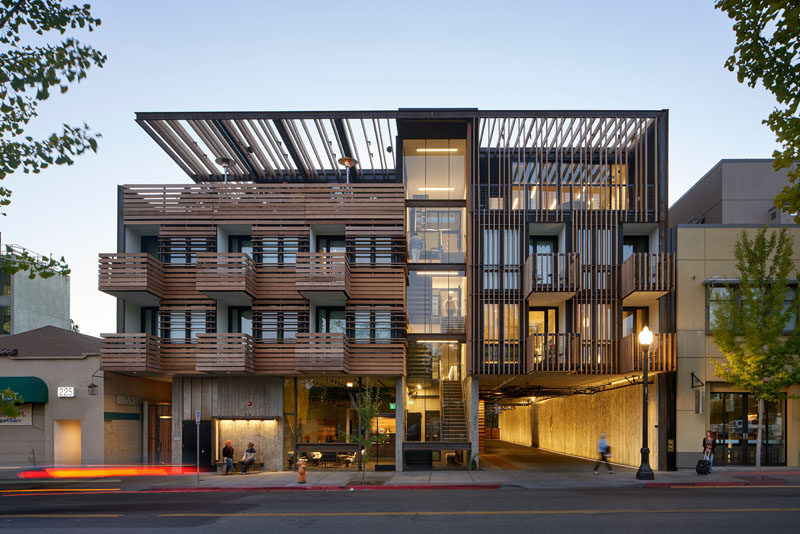The image showcases an outdoor scene under a clear blue sky, featuring a modern building that stands beside a black or gray asphalt road. Flanking the upper left and right corners of the scene are green leafy trees. The building itself is characterized by a sophisticated architectural design with both horizontal and vertical wooden slats adorning the sides and railings. Its middle section is made entirely of glass, displaying staircases that connect each floor. 

On the ground level, there is an entrance to a parking garage at the bottom right corner, with another entrance to the left. A blurred figure walks past, while a lady waits nearby with a luggage bag under the shade of a tree growing from the sidewalk. The building has multiple floors: the ground floor includes the garage and entrance; the next two floors have brownish exteriors, windows, and small patios; and the top floor, visible on the right side, features a long wide window and an expansive terrace with seating and heat lamps under a glass roof with metal slats. An additional awning made of wood extends over part of the building, and another house is visible to its left.